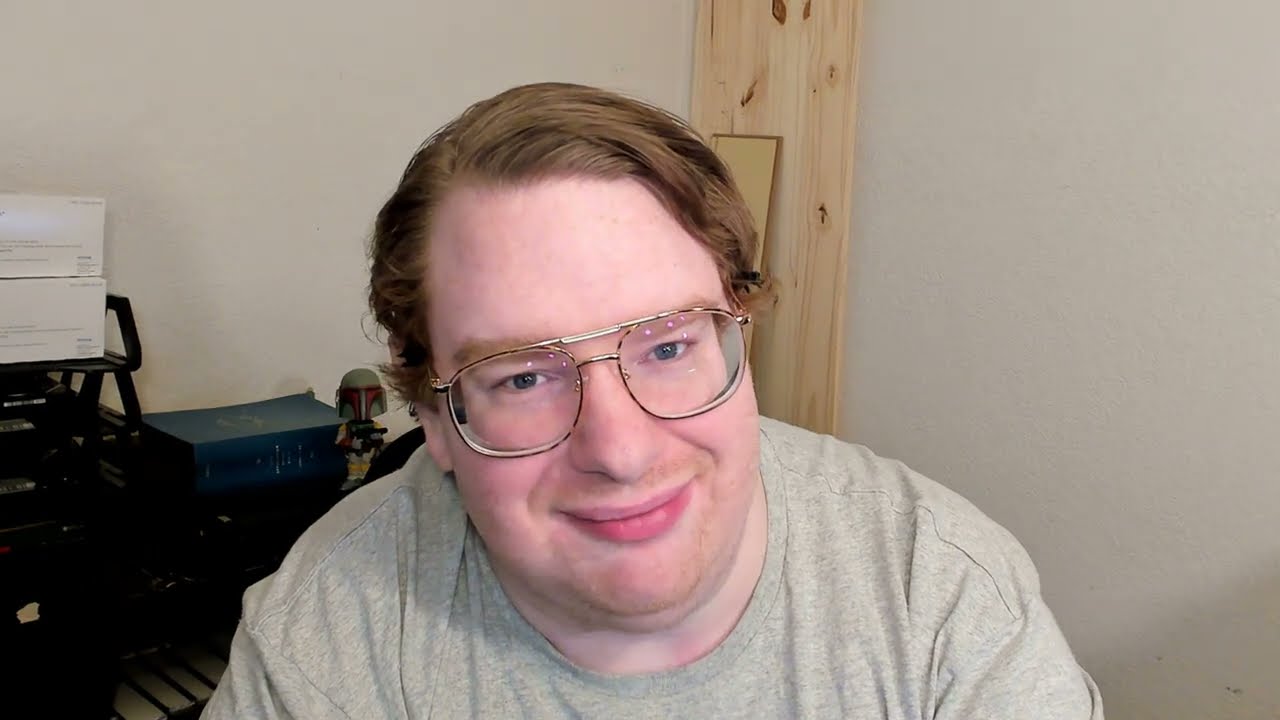In this detailed image, we see a man with a light peach complexion, large gray glasses, and short, reddish-brown hair combed over. He is wearing a light gray t-shirt and is positioned centrally in the photograph, looking directly at the camera with a slight smirk on his face. The backdrop of the image provides a glimpse into his surroundings, suggesting he might be in a home office or a garage.

Behind the man, the wall is plain white with various objects scattered around. To his left, a plank board made of light-colored wood stands vertically. To his right, there is a black desk or trunk-like furniture. On this desk, a blue book is visible along with a colorful bobblehead featuring green, red, yellow, and black hues. Additional details include a shelving unit in the background to his left, which holds some white boxes, and the floor appears to be covered with a rug. The overall scene suggests a casual, somewhat cluttered environment, typical of a personal workspace.